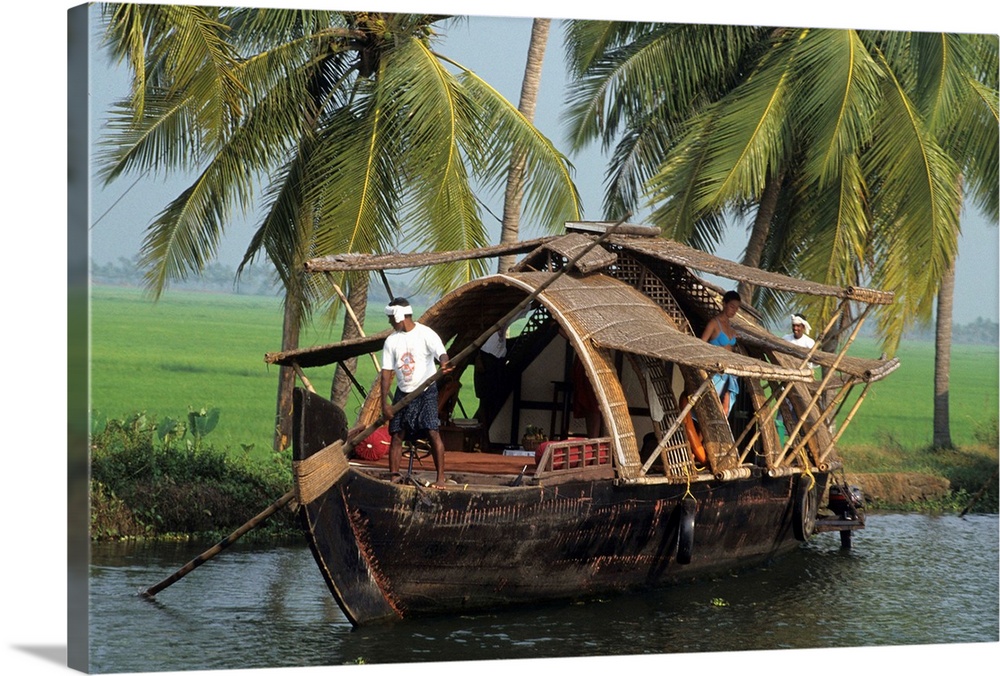The vibrant color photograph captures a scene that appears to be set in the Vietnam area, featuring a detailed and clear depiction of a traditional wooden boat made from wood and bamboo. The boat itself is adorned with a domed roof and a secondary roof that resembles wings. Positioned prominently at the front of the boat is a man clad in a white, short-sleeved t-shirt with a red logo, black swim trunks, and a white headband. He wields a large wooden pole, likely maneuvering the boat. Toward the middle of the vessel, a woman dressed in a blue bikini top and blue denim shorts is seen emerging from the boat's interior. Another man, also in a white shirt, stands at the rear. Surrounding the boat, the landscape is lush and vibrant, with bright green rice fields and palm trees set against a clear, blue sky. The image appears to be a three-dimensional, wrapped canvas print, offering a realistic and immersive view of this serene riverside setting.